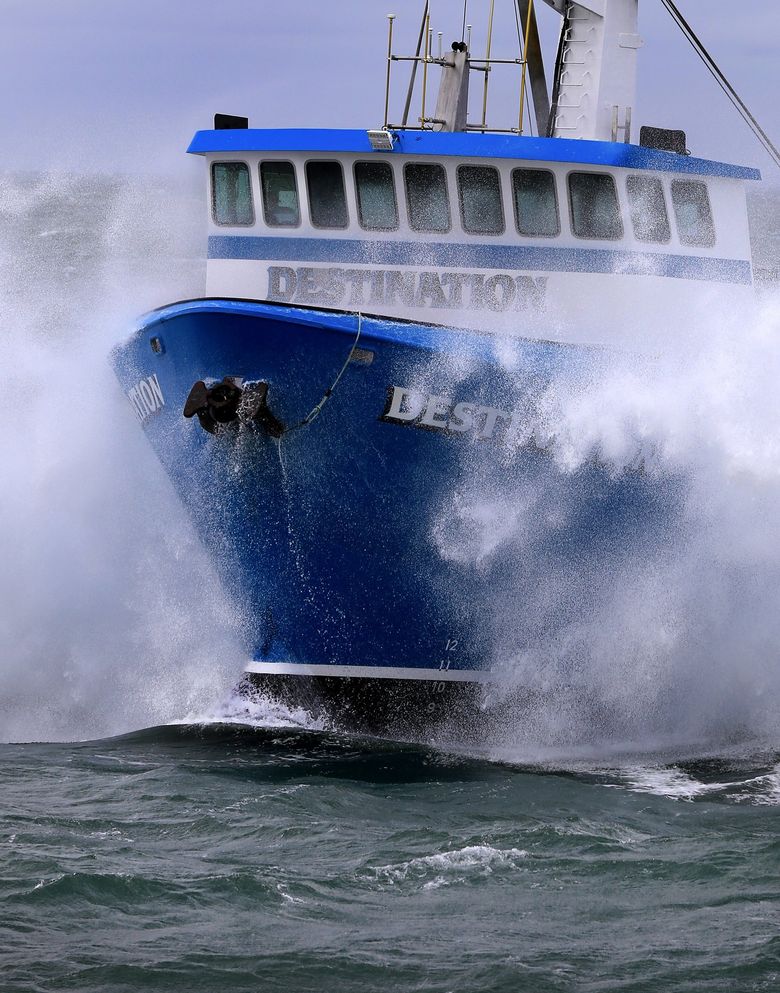The image captures a large blue boat, possibly a ferry, plowing vigorously through deep green waters. The focus is on the boat's frontal view, prominently displaying its bright blue hull and white pilot house adorned with blue stripes and numerous windows. The boat is moving swiftly, creating significant splashes and sprays of water on both sides of its bow. The name "Destination" is partially visible on the pilot house and the side of the hull, with only "D-E-S-T" discernible behind the foaming water. Antennas are seen above the pilot house, hinting at communication equipment. The scene is set on a bright, sunny day with a clear sky, emphasizing the boat's dynamic movement through the presumably oceanic water.